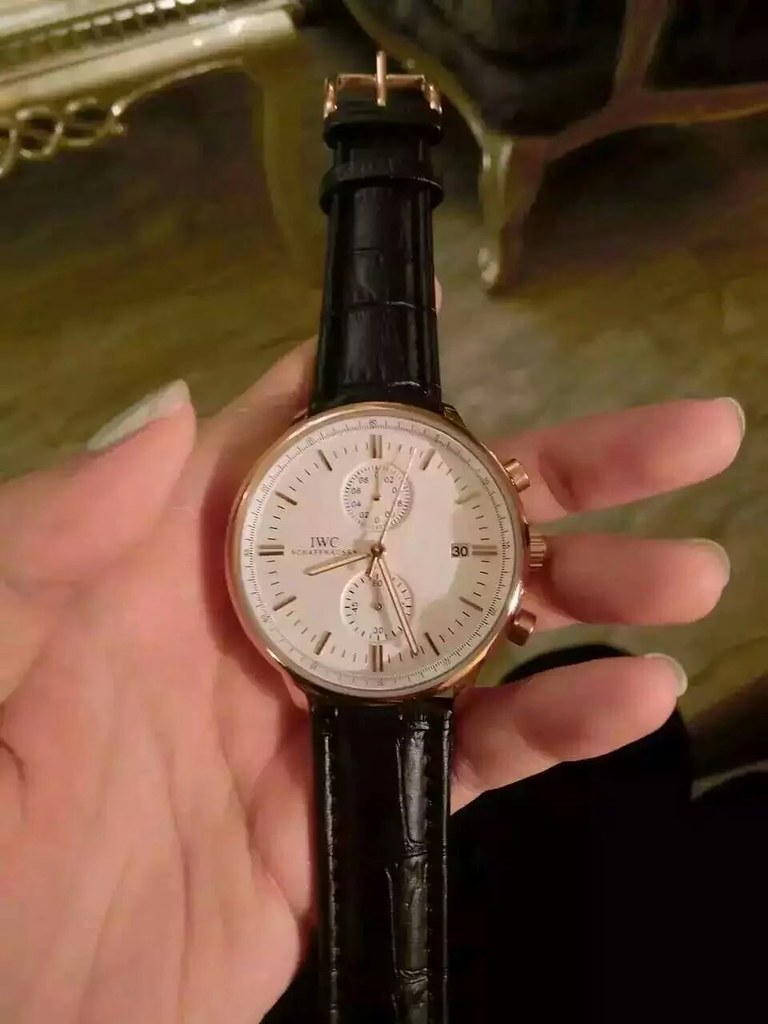The image showcases a luxurious, intricately designed wristwatch held in a person's hand. The watch appears to be of high value, characterized by its detailed craftsmanship that stands out despite its compact size. The timepiece features the branding "JWC" prominently on its face. It includes a date display and possesses two sub-dials situated at the 12 o'clock and 6 o'clock positions. These sub-dials are delicately integrated within the inner circle of the watch face. The hour markers are represented by finely crafted metallic lines, possibly made of gold, adding to the watch's opulent aesthetic. A gold trim elegantly accentuates the periphery of the watch, enhancing its overall grandeur. The person's hand holding the watch shows slightly protruding nails, suggesting that the hand might belong to a female.